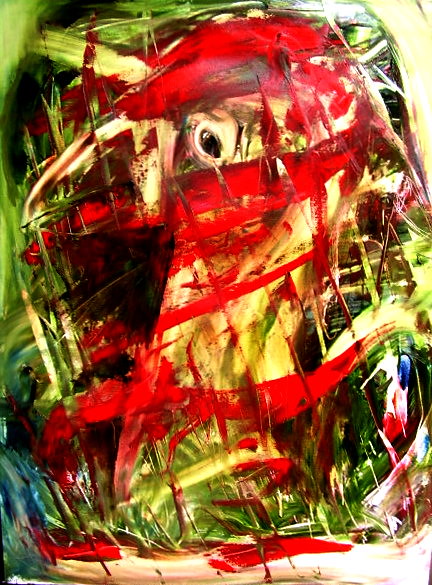This abstract artwork features a central, muddled figure that could be interpreted as a horse, llama, or bird, blending into a chaotic but deliberate composition. The background is primarily black, with patches of green and light brown slashes creating an overcast ambiance. Dominating the center of the piece is a distorted face characterized by a single black eye and an open mouth with a red tongue. Thick red paint splashes across the head, face, and neck of the animal give an impression of blood or injury, adding an unsettling and dramatic contrast.

The lower part of the painting transitions to light blue and white brushstrokes that slant across the bottom, while the rest of the canvas is awash with horizontal streaks of red, green, yellow, and white, evoking a sense of chaotic movement. The artwork, with its generous use of vibrant and dark colors, presents a visceral and somewhat disturbing image, further intensified by the suggestion of a suffering or injured creature. While the portrayal retains enough ambiguity to provoke multiple interpretations, its overall effect is one of intense emotion conveyed through thick, almost haphazard brushstrokes and interspersed vibrant hues.